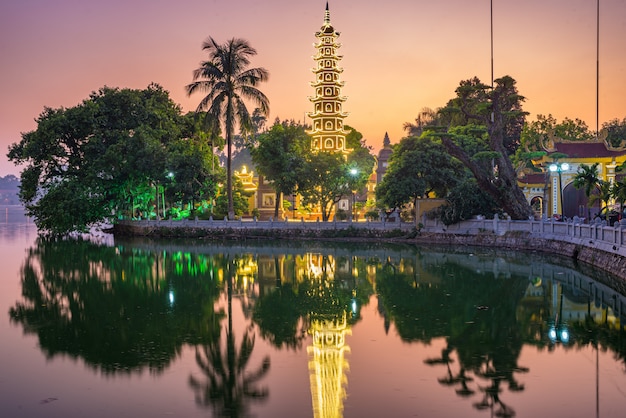The photograph depicts a serene, tropical setting at dusk, with a light pink and lavender sky creating a picturesque backdrop. Dominating the center of the image is a very tall, slender building that resembles a pagoda, adorned with gold lights and topped by a pointed blue ornament. The building's unique spiral design and abundant windows add to its oriental elegance. Surrounding the structure are lush green trees, including large leafy trees and a palm tree to the left. 

In the foreground, a body of water reflects the glowing pagoda and the vibrant sky, adding a sense of tranquility to the scene. The water appears purple and green due to reflections of the sky and nearby vegetation. A cement barrier or pier runs along the middle portion, providing a walkway possibly for visitors to view the water. Additionally, a white fence stretches from the right middle to three-fourths of the way across the scene, marking the boundary between land and water. To the right are a few white buildings nestled among the trees, enhancing the postcard-perfect charm of this tropical locale.